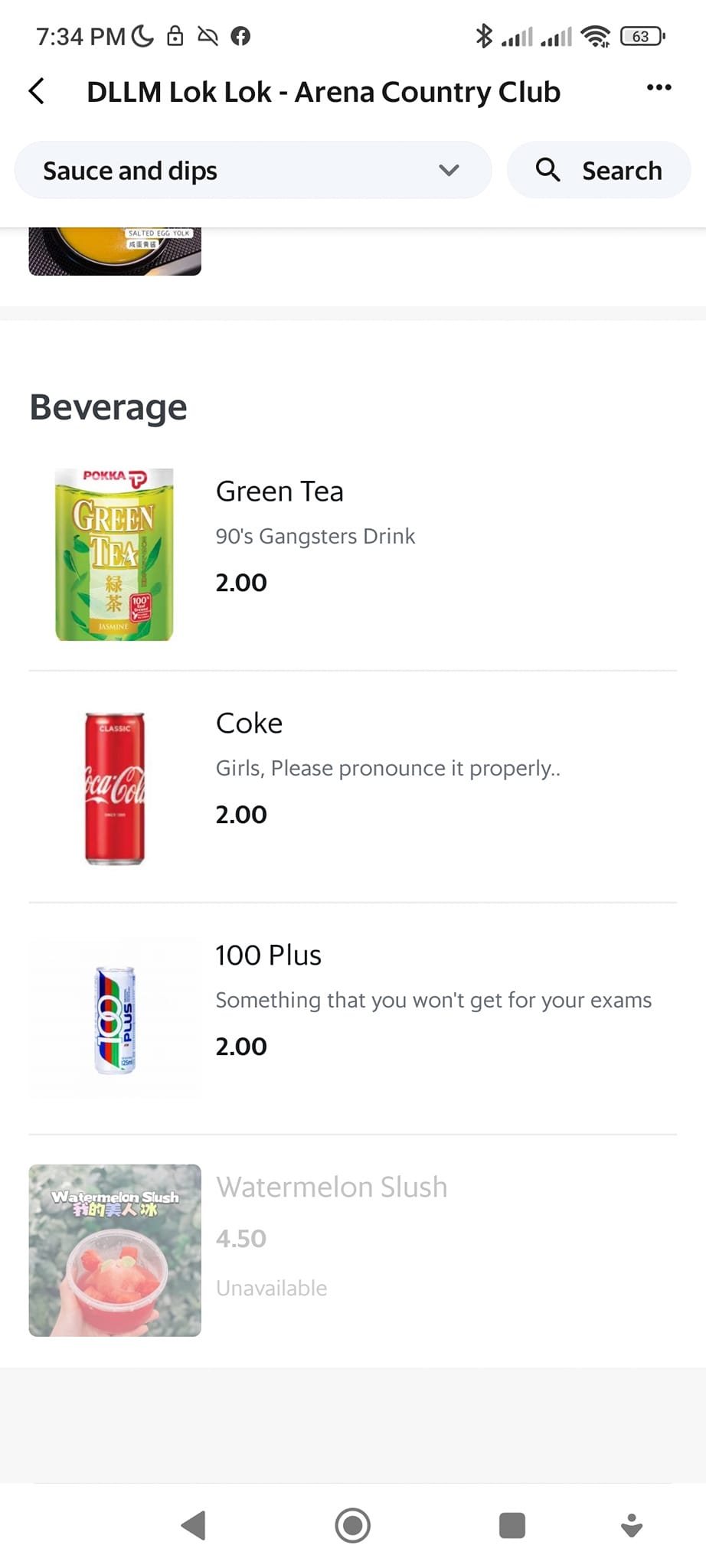This screenshot captures a detailed view of a cell phone screen displaying a menu interface against a white background with black and gray text at the top. 

In the top left corner, the time reads 7:34 PM, accompanied by a moon icon indicating night mode. Adjacent to these, there is a series of icons: a lock icon, an icon resembling a crossed-out cloud, and a Facebook icon. Meanwhile, the top right corner showcases icons for Bluetooth, reception bars, Wi-Fi, and a battery level at either 63% or 68%. 

A left-pointing arrow and the text "D-L-L-M, lock, lock, Urbina Country Club" appear immediately below this. A drop-down menu offering selections of sauces and dips resides next to a search bar. 

The main section reveals part of a drink menu. Heading this menu is a partially cut-off header, followed by a clear label: "Beverages." The menu presents three items:

1. **Green Tea**: Featured with an image of a green tea container, its description reads "90s gangster's drink," and it is priced at $2.
2. **Coca-Cola (Coke)**: Accompanied by an image of a Coke can, the listing advises, "Girls, please pronounce it properly," with a price of $2.
3. **100 Plus**: This listing humorously notes that it's "something that you won't get for your exams," also priced at $2.

The screenshot encapsulates the quirky and humorous descriptions of the drink offerings at Urbina Country Club, providing both practical information and a touch of personality in its layout.